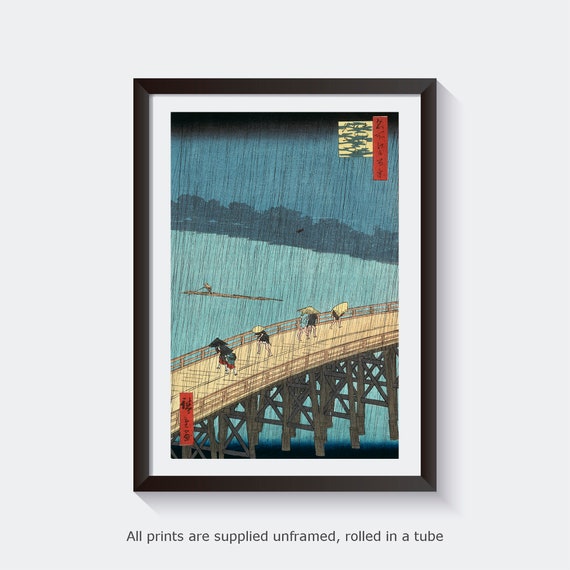This is an artistic print displayed in a black frame with a white mat, mounted on a flat white wall. The inscription at the bottom of the frame reads, "All prints are supplied unframed, rolled in a tube." The framed print captures an evocative, possibly Japanese, scene dominated by a bridge extending over a river, upheld by wooden posts. The setting is characterized by heavy rainfall, with several individuals crossing the bridge, all sheltering under umbrellas or hats. In the distance, a man maneuvers a long boat with an oar. The print also features red upright banners with Japanese lettering in the upper right and lower left corners. Hints of beige, brown, blues, and a touch of red enhance the atmospheric quality of the rainy scene, set against a somewhat indistinct backdrop of trees, land, or mountains.